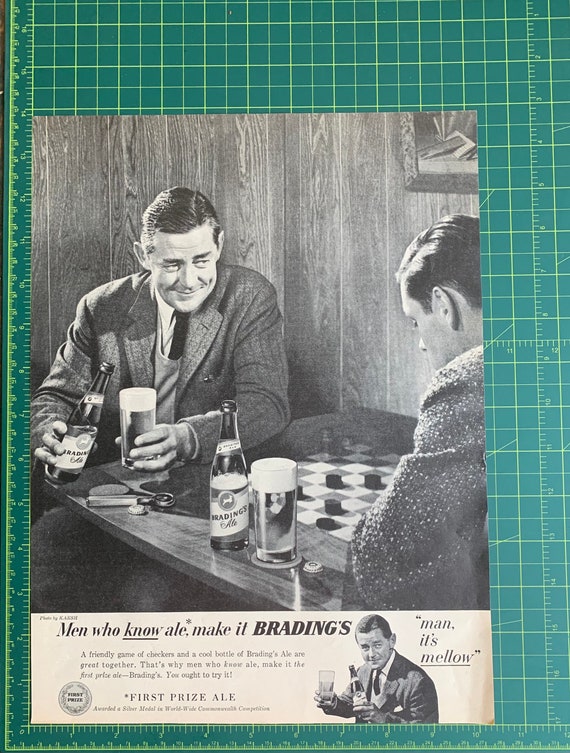The image features an old black-and-white magazine advertisement, likely from the 1920s, set against a green cutting board with a grid of measurements, giving it the appearance of trying to measure the ad. The advertisement showcases two men sitting at a table, engaged in a game of checkers. Each man has a bottle and glass of Brading's Ale in front of him. The man facing the camera is pouring a beer, while the other is contemplating his next move. The tagline at the bottom of the ad reads, "Men who know ale, make it Brading's." Another line in the ad quotes one of the men saying, "Man, it's mellow." The ad also features an emblem indicating that Brading's Ale is a first prize winner. The nostalgic scene and detailed depiction suggest a leisurely moment, combining the pleasures of a friendly game and a good ale.